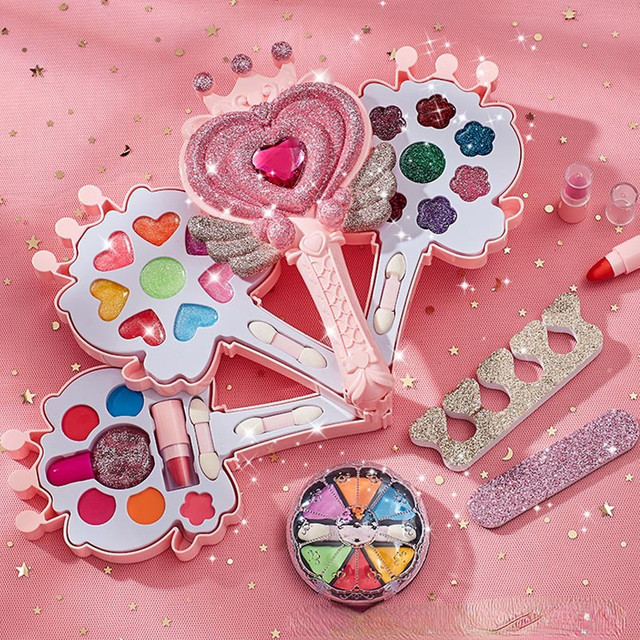The image depicts a lively, vividly pink setup, likely a party scene aimed at young girls. The foreground features a shiny pink tablecloth adorned with glittering confetti in the shapes of stars, circles, and hearts, contributing to the festive atmosphere. Centered on the tablecloth is a charming makeup set that resembles a magical wand, complete with a heart symbol adorned with wings at the top. This layered makeup kit unfolds to reveal various compartments containing an assortment of cosmetics, including nail polish, lipstick, and small applicators. The setup also includes a toe separator, indicating that the kit is intended for nail care and makeup fun. The entire display is sprinkled with digital sparkles, enhancing its enchanting and whimsical appearance, perfectly suited for a young girls' party.